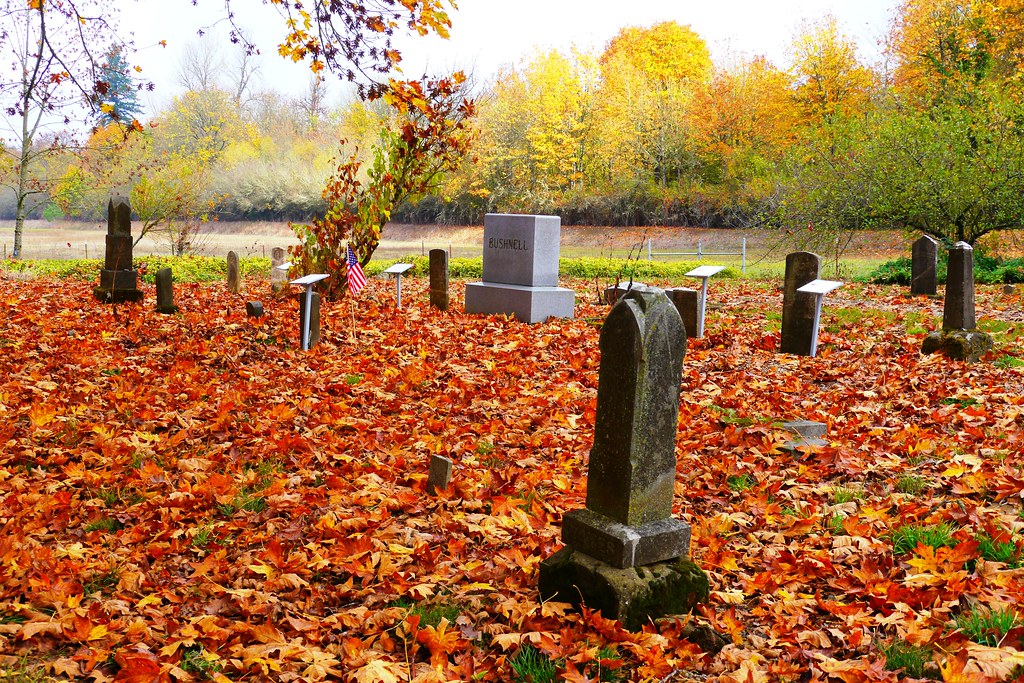The photograph captures a somber, autumnal scene in an old graveyard. The ground is completely covered with a dense blanket of red, yellow, and brown leaves, obscuring the grass beneath. Among the assorted weathered gravestones—many of which are dark gray, moss-covered, and aged—there stands one prominently modern, clean, and polished granite headstone inscribed with the name "Bushnell." Adjacent to a smaller headstone on the left side of the image, an American flag is staked into the ground. The backdrop features a forest of trees transitioning through their autumnal hues of green, yellow, and orange, reinforcing the cycle of life and death symbolized by the fallen leaves. Some of the gravestones display a brownish, mildewed texture that marks their antiquity. The entire scene, devoid of any people, emanates a melancholic and reflective atmosphere, accentuated by the seasonal transformation of the surrounding nature. In the far background, there is a glimpse of a little creek or river, adding a soft, flowing element to the otherwise still and silent graveyard.